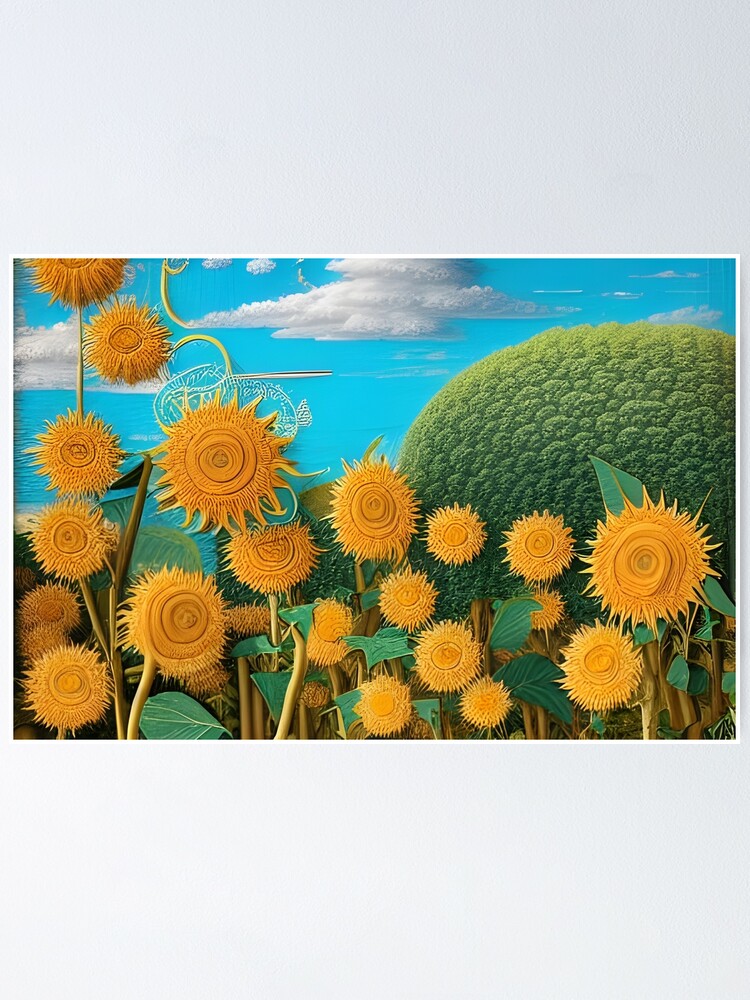This is a computer-generated image depicting a whimsical and futuristic sunflower field under a bright blue sky with white and gray clouds. In the foreground, around 15 to 20 mustard-orange sunflowers with circular petals and swirling centers fill the scene. These sunflowers have orange and yellow-brown stems and green leaves, giving them a fantastical appearance reminiscent of actual suns. The background features a large, cartoonishly shaped tree, its rounded, densely packed greenery resembling a crown of broccoli, extending off the right edge of the image. At the top of the image, some sunflowers appear to float into the sky, their stems curling around them, adding to the dreamy, playful aesthetic of the artwork.